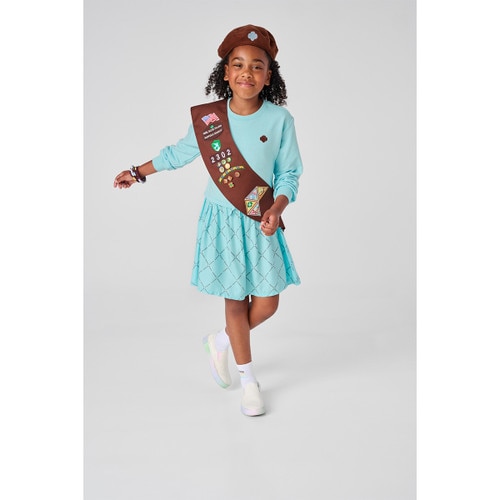In this detailed image, a young Girl Scout, likely around 5 to 6 years old, stands prominently in the center. She sports the distinctive brown uniform of a Girl Scout, complete with a brown dungaree-style dress with overall snaps and a matching beret-like hat. Underneath her uniform, she wears a white t-shirt lined with a blue trim. Draped across her chest is a sash adorned with numerous achievement badges, including an American flag and the number "373," as well as the inscription "Girl Scouts USA."

She has her hair braided into pigtails and beams widely, her hands clenched gently at her sides. The setting appears to be a Girl Scout event; she stands in front of a table covered with a teal green tablecloth. On the table, there are various items, possibly baked goods, indicating they might be for sale. Behind the table is a woman whose head is out of the frame. The woman is dressed in a purple t-shirt and a blue zip-up vest. The background reveals some blurred greenery, suggesting the event is taking place outdoors or in a park-like area. The overall cheerful and organized scene reflects a moment of pride and accomplishment for the young Girl Scout.